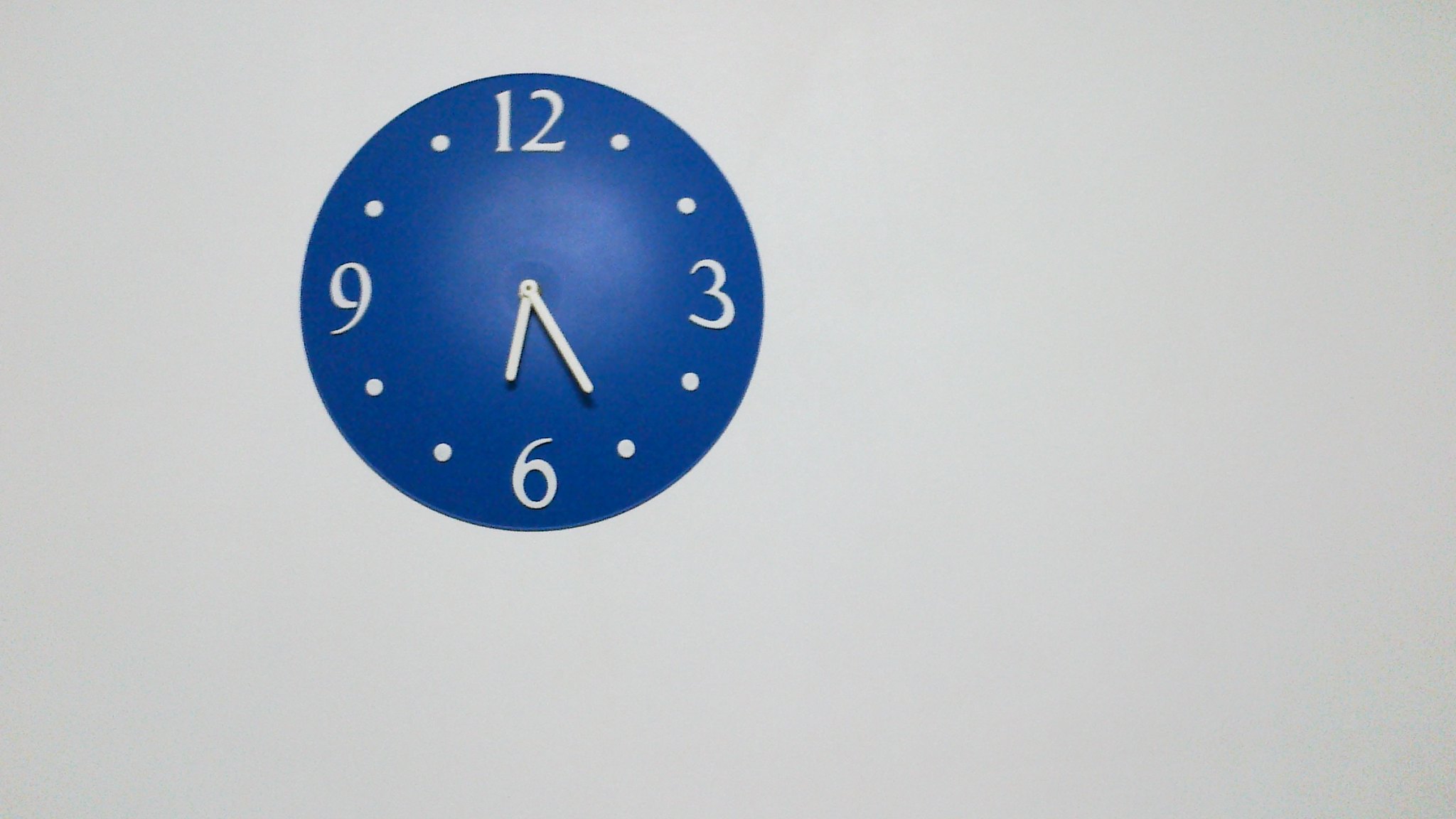The image features a minimalist blue clock set against a plain white or possibly pale gray background. The clock face is a simple blue circle that gradually lightens towards the center, creating a subtle gradient effect. Bold white numbers mark the 12, 3, 6, and 9 positions, while small white dots represent the other hours. The clock hands, also white, indicate the time as 6:25. The clock is positioned slightly towards the upper left within the frame, lending an impression of asymmetry. The overall aesthetic is clean and simplistic, suggesting it may be a high-quality photograph or a digital graphic, possibly intended for a modern interior design catalog or a minimalist art display. The nuanced fade of blue and clear depiction of details make it appear almost like a stylized studio shot or a digital creation resembling a real clock.